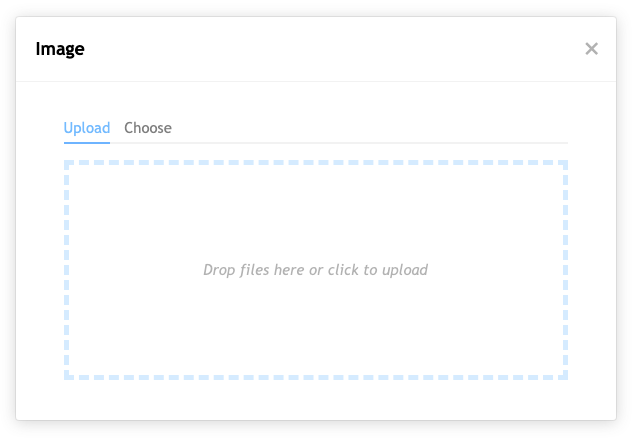This image depicts a file uploading interface on a web page. In the top left corner, the label "Image" is displayed in black text. Opposite to it, in the top right corner, there is a grey-colored "X" button. Below the header, there are two options: "Upload," which is written in blue and underlined, and "Choose," which is written in grey. Dominating the center of the interface is a large blue rectangular box, outlined with blue broken lines. In the center of this box, there is a grey text prompt that reads, "Drop files here or click to upload." Overall, this webpage is designed to facilitate the uploading of files.